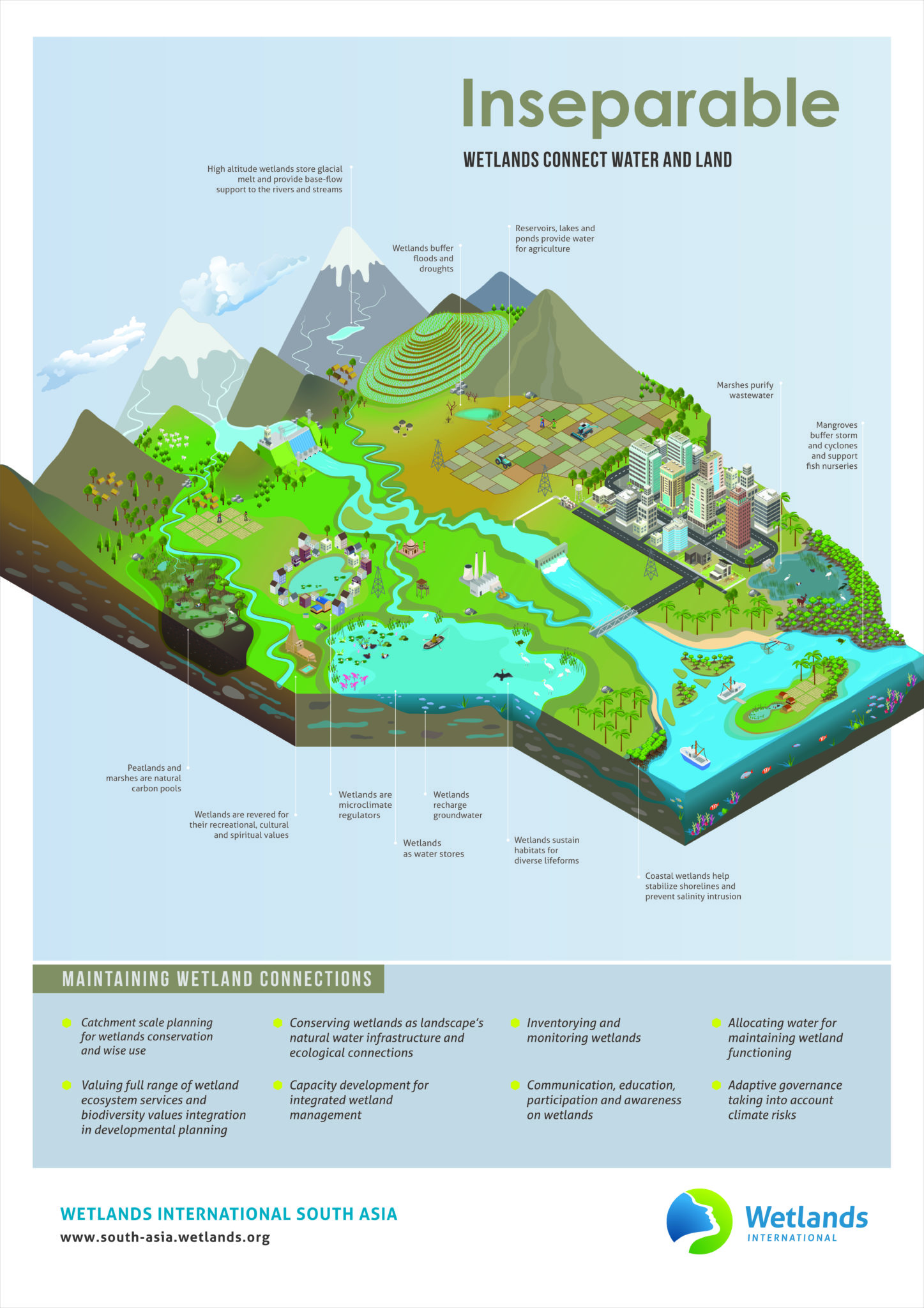The poster vividly illustrates how wetlands serve as the critical link between land and water, utilizing a detailed drawing. At the top right corner, the word "inseparable" is prominently written in green, with the phrase "Wetlands connect water and land" in bold black beneath it. The image depicts water flowing from the mountains on the upper edge of the map, cascading through a diverse landscape that includes a bustling city, expansive farmland, terraced rice fields, and serene ponds. This depiction emphasizes the interconnectedness of urban and rural environments through the wetlands.

Towards the bottom, the words "maintaining wetland connections" stand out, with informative sentences below outlining strategies for wetland conservation and sustainable use. These include "catchment scale planning for wetlands conservation and wise use," "valuing the full range of wetland ecosystems," "conserving wetlands as landscapes, natural water infrastructure, and ecological connections," and "capacity development for integrated wetland management." Additionally, the text highlights the importance of "inventory and monitoring wetlands," "communication, education, participation, and awareness," "allocating water for maintaining wetland function," and "adopting governance to address wetland climate risks."

Despite some of the text being too small to read clearly, the poster's visual and readable elements effectively convey the message that wetlands are vital for connecting land and water, highlighting their ecological, infrastructural, and societal importance.